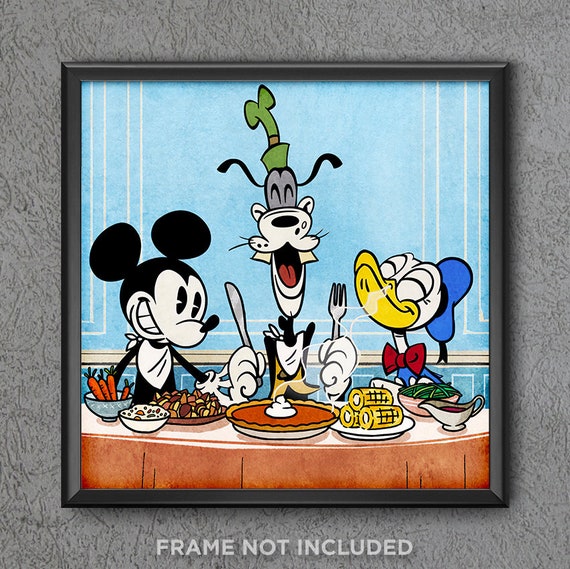The image is a detailed cartoon artwork featuring Mickey Mouse, Goofy, and Donald Duck, reminiscent of vintage Disney designs akin to "Steamboat Willie," though presented in color. The trio is seated around a reddish-orange table covered with a variety of foods including carrots, green beans, corn, a pie, nuts, and gravy. Mickey is positioned on the left with a broad, toothy grin; Goofy is in the middle, exuberantly holding a fork and knife with a big smile on his face; and Donald is on the right, lifting his beak and enjoying the aroma of the pie. The background of the image is a muted blue, contrasting with the vibrant colors of the characters—Goofy's green hat, Donald's blue outfit with a red bow tie, and the various hues of the food. This framed artwork is captioned "frame not included" at the bottom, suggesting it is a purchasable item. The characters are all depicted with napkins tied around their necks, eagerly anticipating their meal, which adds a touch of whimsy and delight to the scene.